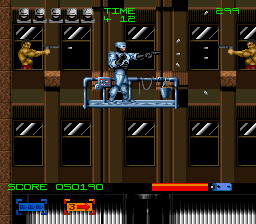The image, a screenshot from a video game, depicts an intense action scene set against the backdrop of a dark and light brown brick business building with black windows, outlined by dark and light gray lines to simulate reflections. Prominent features include a blue-silver scaffolding platform used by window washers, on which stands a robot-like figure, possibly a "robocop," armed with a black gun. He aims to the right, where a shirtless man in red pants, also armed, aims back at him from a window. Mirroring this setup, another shirtless man in red pants leans out of a window on the left, also targeting the robot man. The game interface displays various elements in red, blue, and green fonts, including "Time 4-12-299" and a green score at the bottom. At the top of the screen, icons resembling army heads indicate lives or remaining time, adding to the adrenaline-fueled atmosphere of this side-scrolling shooter game.